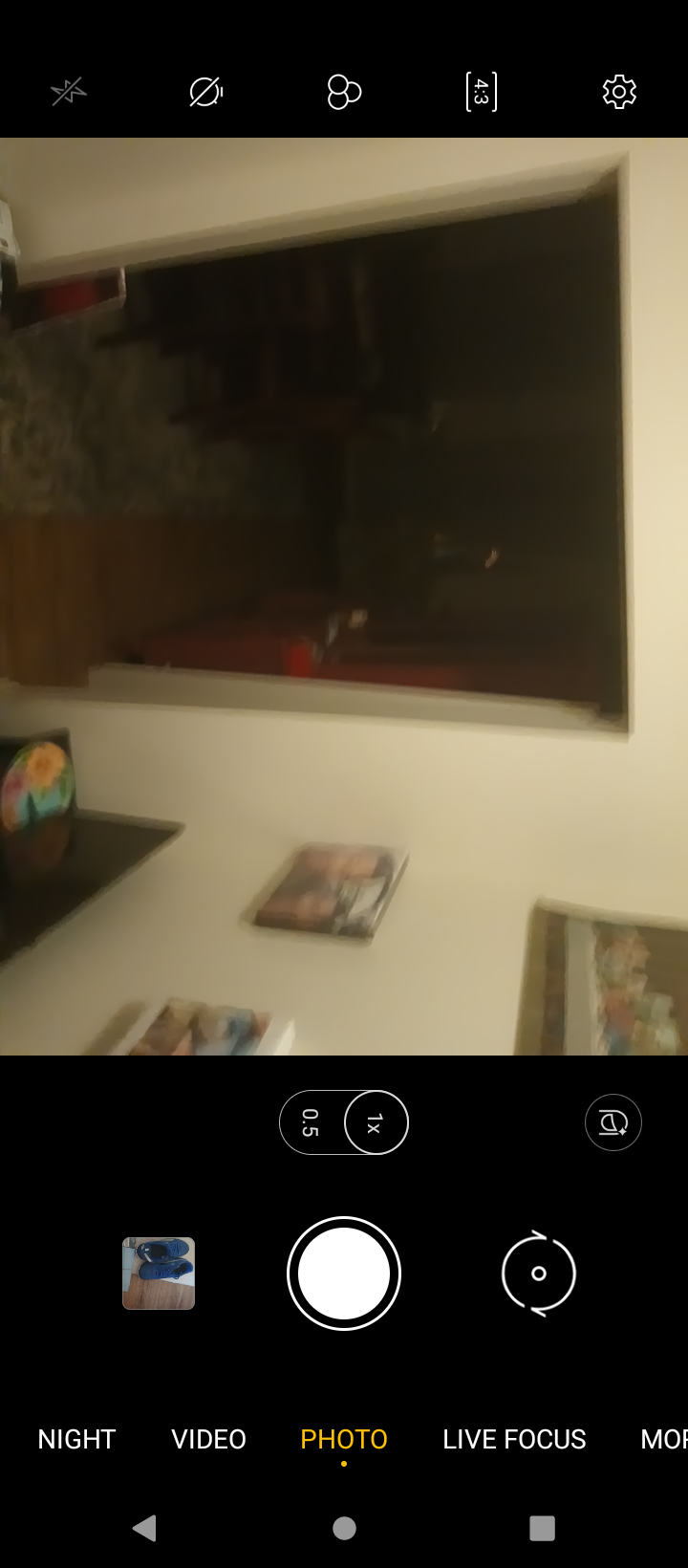This image is a screenshot taken from a phone's camera app, evident from the on-screen options like "night," "video," "photo," and "live focus" displayed at the bottom. The interface shows the no-flash icon, a no-timer or filter indication, ratio settings, and additional settings at the top. The image within the screenshot captures the inside of a house, specifically from the foyer area. A bench is positioned beneath two small pictures and a larger one above them on an off-white wall. The view extends into a darkened room through a doorway, where a piece of red furniture is visible to the right and another brown item is discernible to the left, though details remain obscured due to the room's darkness. The camera interface also shows a selected 1x zoom on the bottom, accompanied by a big white shutter button and various camera mode options, indicating the comprehensive nature of this screenshot within a house interior scene.